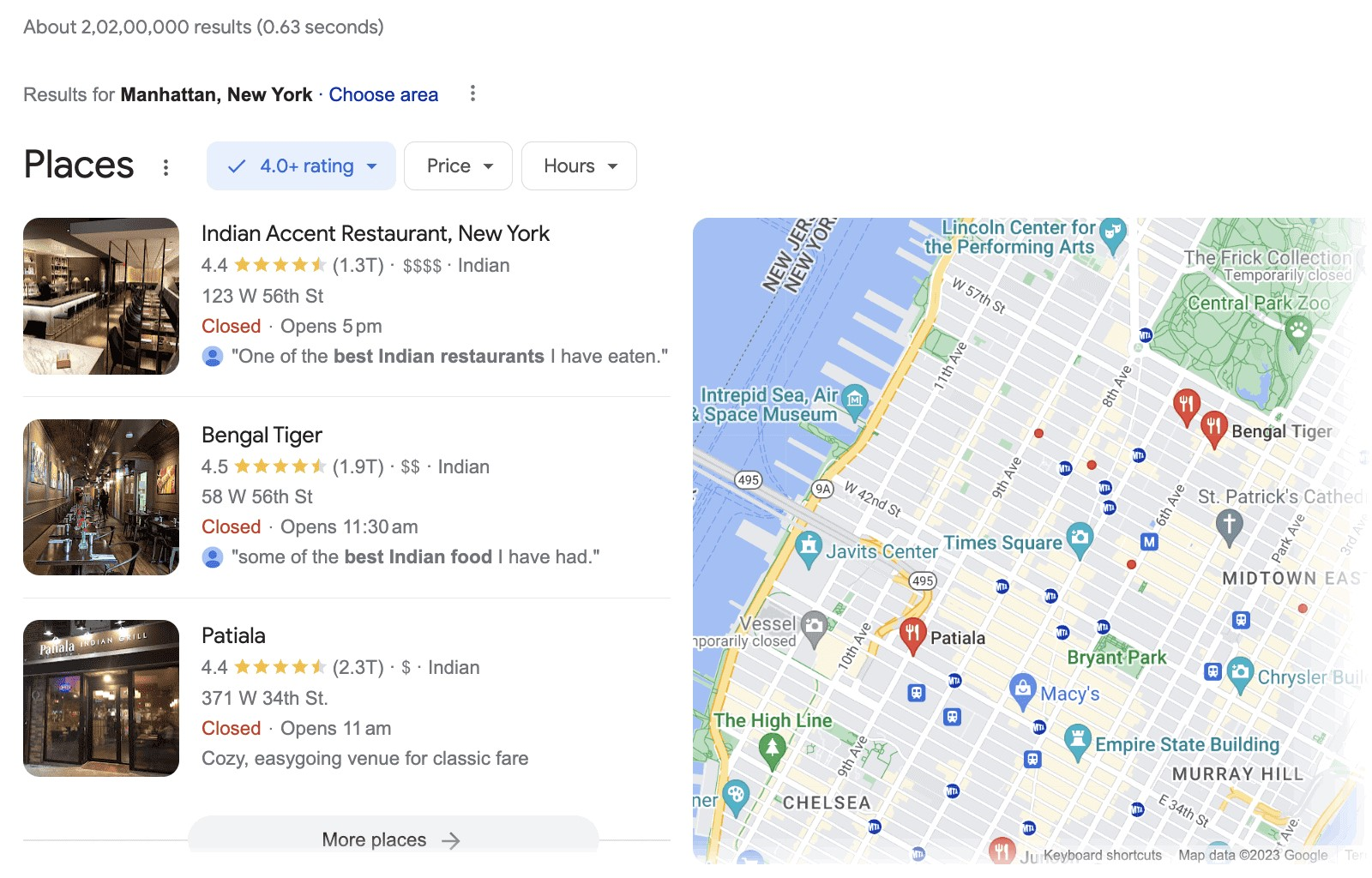This is a detailed screenshot from Google Maps displaying search results for restaurants in Manhattan, New York. The right side of the screenshot features a bird's eye view map highlighting the cityscape with various landmarks, including gray buildings and the characteristic red pinpoints denoting restaurant locations. These pinpoints indicate the search focus is on restaurants. Light blue droplets identify tourist attractions. The map also displays the signature blue, red, and yellow colors associated with the Google Maps logo.

On the left side, the search details are provided. At the top, the search information indicates approximately 2,202,000,000 results were found in 0.63 seconds. It specifies the search area as Manhattan, New York, and offers the option to refine the search area. Below this, filtering options are available, with criteria such as rating (4.0+), price, and hours of operation. The 4.0+ rating filter is highlighted in blue.

Three restaurant entries are visible in the search results. Each entry includes a thumbnail image of the restaurant on the left and detailed information on the right. The first entry is for "Indian Accent," a restaurant in New York with a 4.4-star rating, located at 123 West 56th Street, and marked as currently closed. A quote underneath mentions, "One of the best Indian restaurants I've eaten." The second entry is for "Bengal Tiger," while the third is for "Patiala." Specific details about the ratings, addresses, and statuses for these last two restaurants, however, are not fully visible in the screenshot.